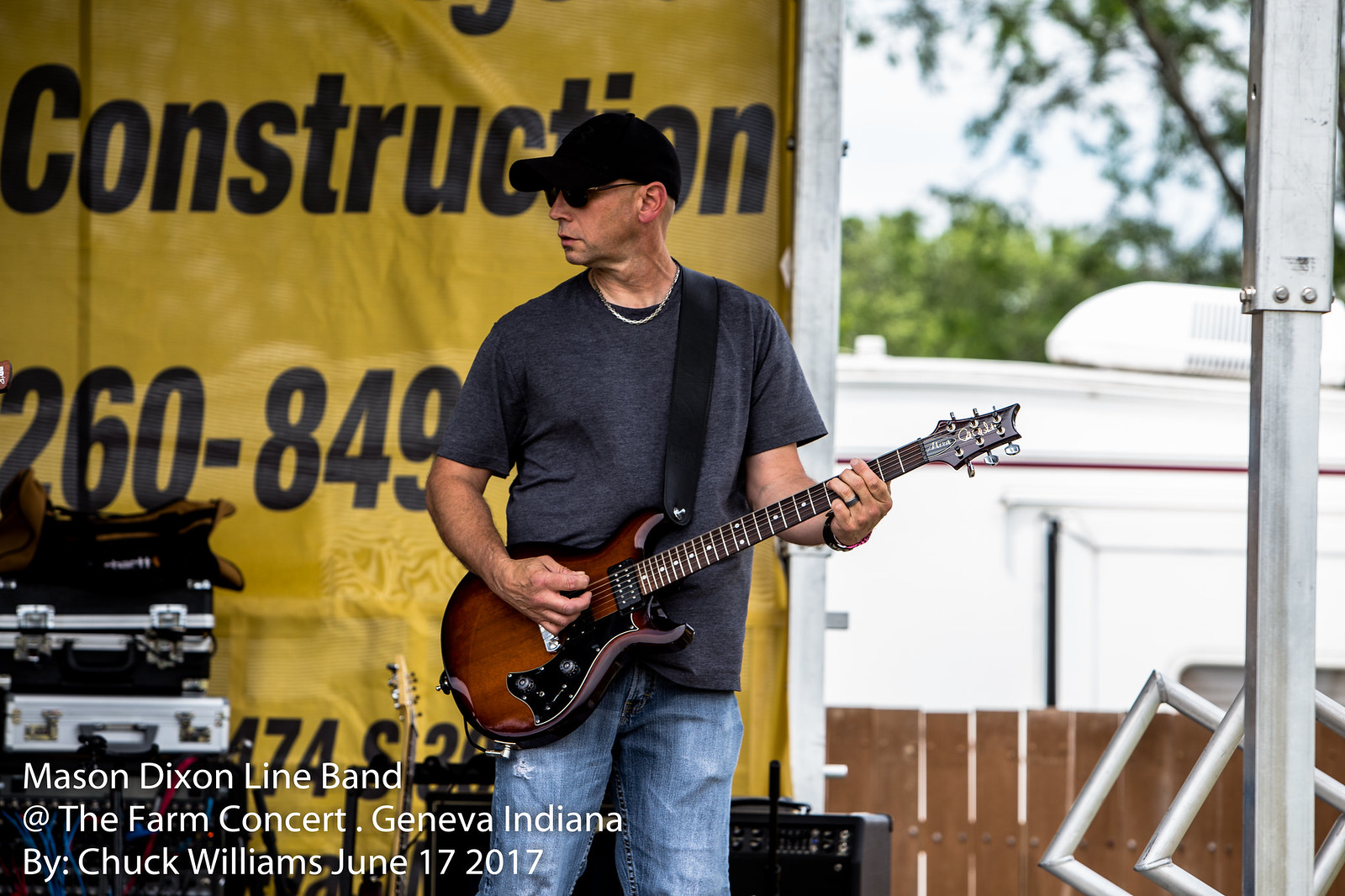This photograph captures a middle-aged white man, likely in his 50s, performing on stage at the Farm Concert in Geneva, Indiana, on June 17, 2017. He is a member of the Mason Dixon Line Band. The man is playing an electric guitar, which has a stained wooden finish, supported by a strap over his shoulder. He is dressed in a gray t-shirt and blue jeans, accessorized with a small chain necklace. He also wears a black baseball cap and sunglasses, and is clean-shaven. His body faces forward while his head is tilted, looking off to the left. In the background, a white banner with the word "Construction" and some numbers is visible, which appears to be part of some advertising. Additionally, there is a trailer or camper positioned behind a fence to the right. The bottom left corner of the photograph features white text that reads, "Mason Dixon Line Band at the Farm Concert Geneva, Indiana by Chuck Williams, June 17, 2017."